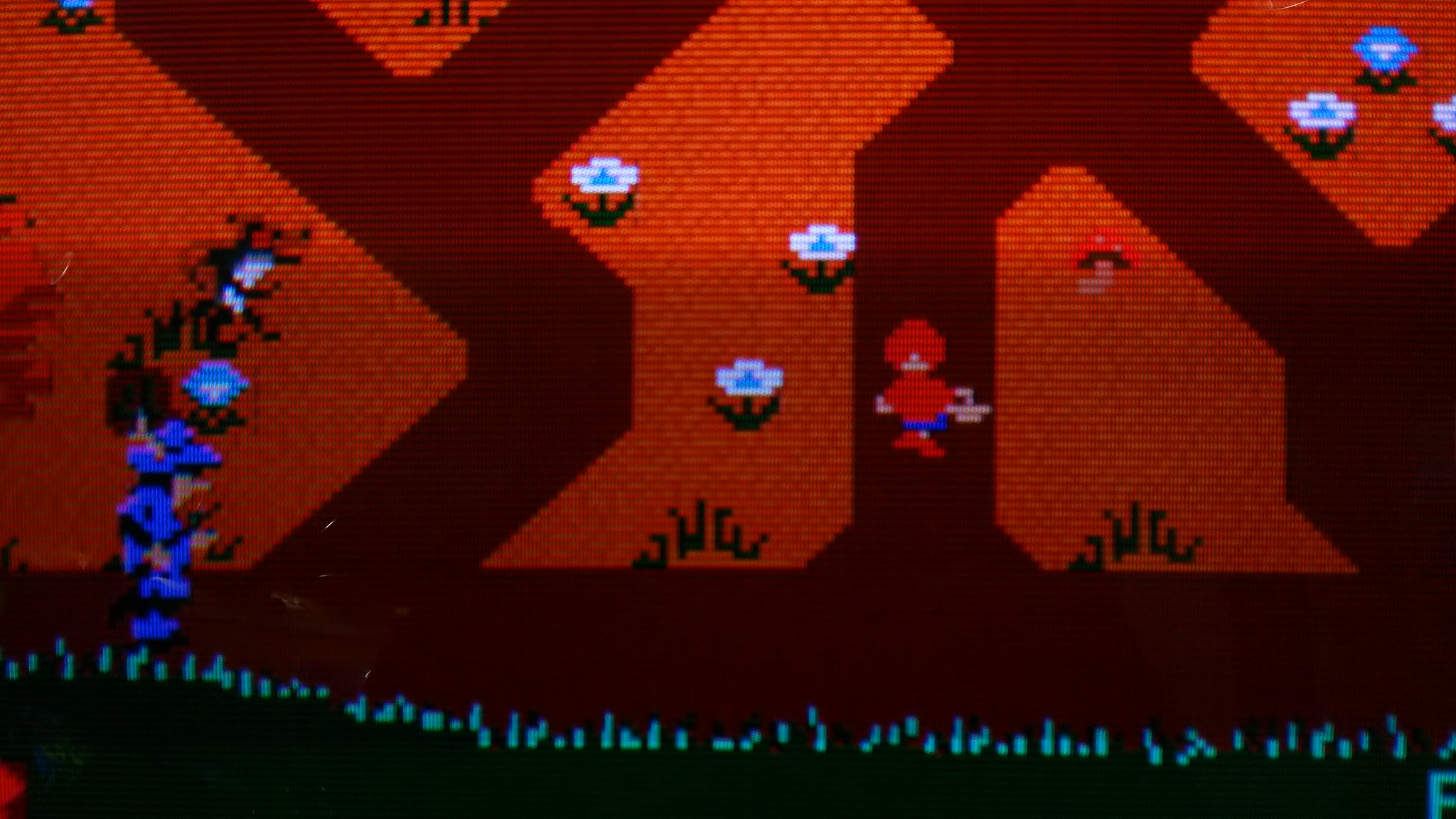The image appears to be a photograph of a computer or TV screen displaying an 8-bit vintage video game, reminiscent of an Atari 2600 title. The graphically simple and pixelated design features a predominantly reddish-orange background with darker brown pathways and greenish-bluish elements intended to represent grass across the bottom of the screen. On the left side of the image, there's a figure dressed in blue, carrying an object, possibly a basket or picnic item. In the center of the scene, geometric landmasses are adorned with flowers, a mixture of which are white with blue centers. Towards the right-hand side of the screen, another figure, sporting a red hat, red shirt, blue skirt, and red shoes, appears to be walking away from the screen, also carrying a basket. The overall scene is completed with additional pixelated flowers scattered, including a blue one and a couple more white ones in the top-right corner.